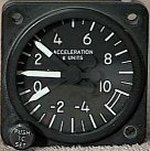The image depicts a compact, square-shaped measuring device resting on a soft surface, possibly a beige or gray carpet. At the center of the device is an elevated circular rim resembling a clock face, but instead of displaying time, it appears to measure pressure. The face features a unique arrangement of numbers: 6, 8, 10, -4, -2, 0, 2, and 4, with lines replacing traditional positions like 12 o'clock. Notably, the device has three hands instead of the conventional two found in a clock. The corners of the square frame have small holes, designed likely for screws to attach the device to another surface.